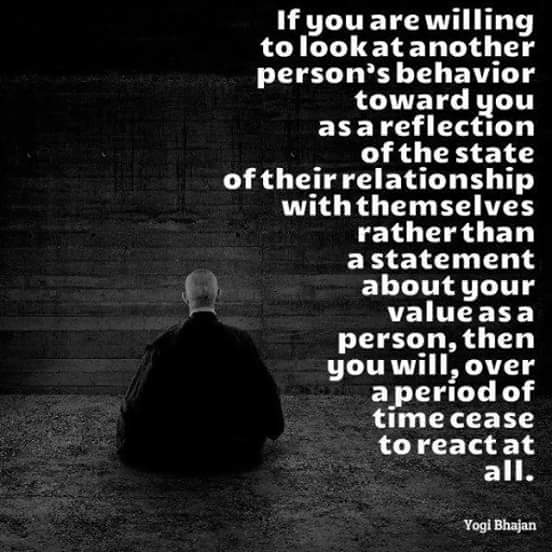This black-and-white square image features a powerful motivational quote by Yogi Bhajan. The text, in white lettering running down the right side, reads: "If you are willing to look at another person's behavior toward you as a reflection of the state of their relationship with themselves, rather than a statement about your value as a person, then you will, over a period of time, cease to react at all." On the left side of the image, a bald man is seated on a carpeted surface with his back to the camera, staring at a wooden wall. He is dressed in dark, possibly black clothing, which includes a shroud or cloak-like garment, and a white collar is faintly visible. The image's monochromatic scheme lends a contemplative and serene atmosphere, enhancing the reflective nature of the quote.